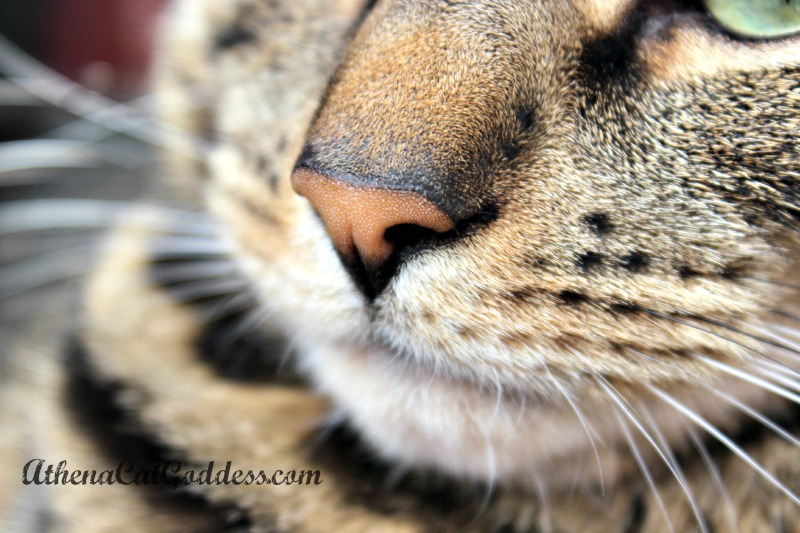This image is an extreme close-up macro shot of a tabby cat's face, capturing intricate details of its nose, whiskers, and partial eye. The nose of the cat is a pale salmon color with a slightly darker top. The cat's white whiskers spring prominently from its nose and chin, contrasting with the fur, which varies in color from black to shades of orange-brown and beige. The image showcases the textured stripes across the cat's chest. In the upper right corner, part of the cat's green left eye is visible, likely around 30% of it due to the close-up nature of the shot. The bottom left corner of the image contains partially obscured text in black cursive, reading AthenaCatGoddess.com. This detailed photograph emphasizes the cat's distinct features and texture.